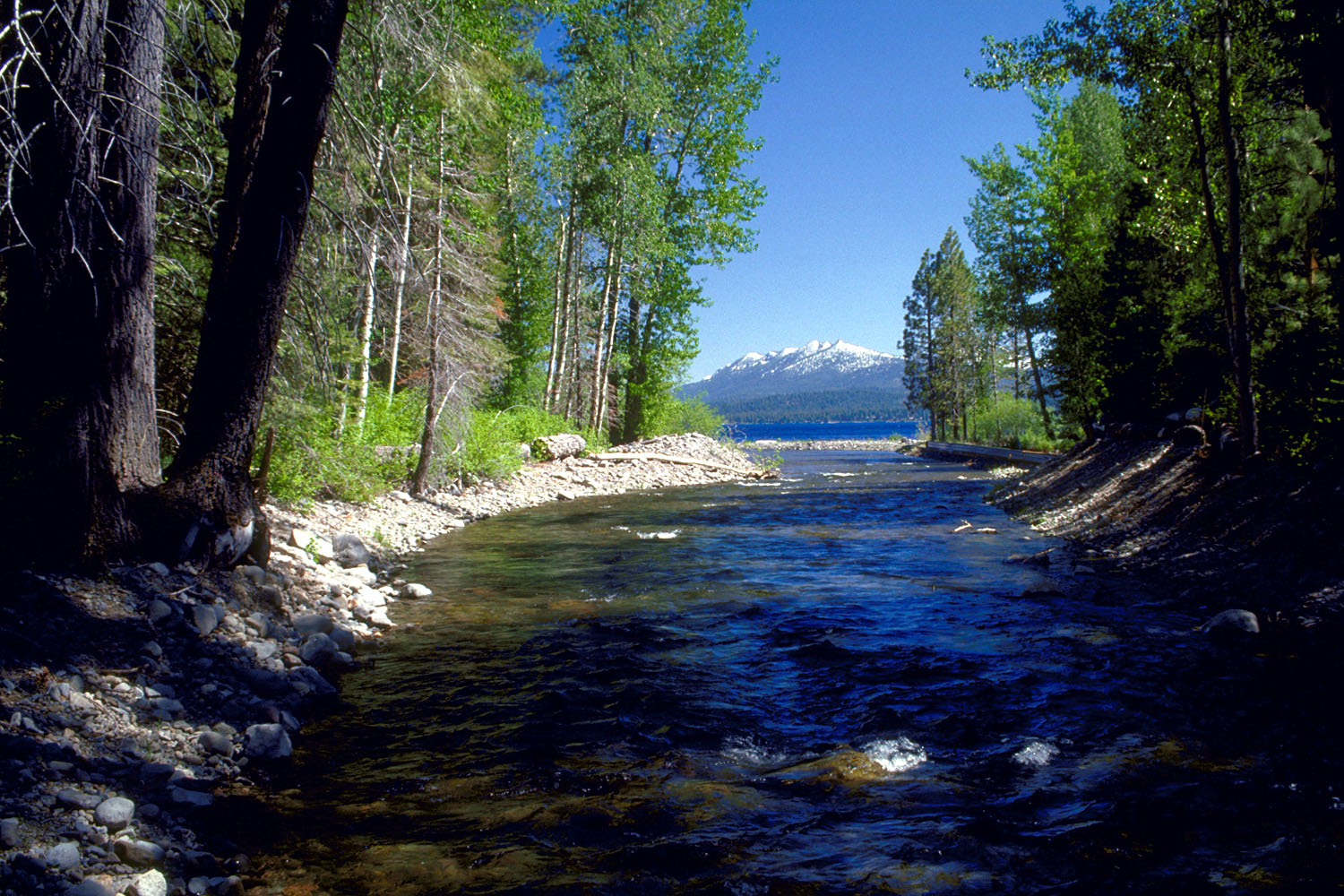A picturesque waterway, larger than a stream but smaller than a river, flows energetically through a varied landscape. On the right bank, an array of rocks is scattered along the shore, possibly deposited by the swift currents that characterize this body of water. To the left, a dense collection of trees lines the shore, where the terrain gently ascends into a gradual slope, perhaps shaped by fluctuating water levels over time. The rapid flow, dotted with protruding rocks, suggests potential for beginner-level whitewater rafting. The waterway, lively and turbulent, continues its journey toward a vast body of water visible in the distance. Towering above this serene scene is a majestic, snow-capped mountain, its base cloaked in lush forest. The snow-covered peak adds an imposing yet tranquil backdrop to the flowing waters, which appear to have sculpted the rocky shoreline.